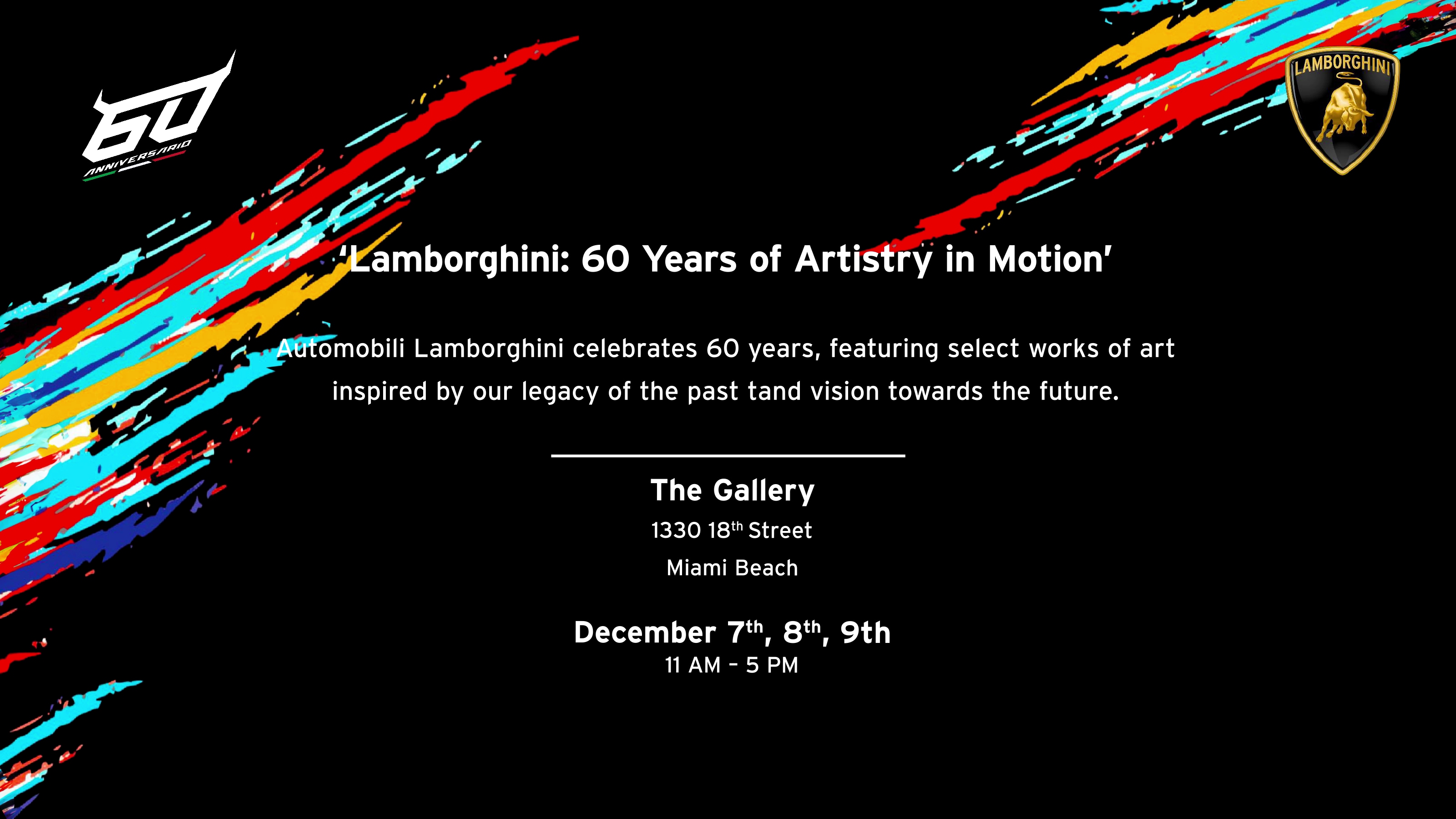The advertisement, with a sleek black background, prominently displays in white text, "Lamborghini, 60 Years of Artistry in Motion." It celebrates Automobile Lamborghini's 60-year legacy, showcasing select works of art inspired by their past and vision for the future. Highlighting the event details, it announces an art exhibit at The Gallery, 1330 18th Street, Miami Beach, on December 7th, 8th, and 9th, from 11 a.m. to 5 p.m. In the top left corner, the number "60" marks the anniversary, while the top right features the iconic Lamborghini logo—an upside-down triangle with a poised golden bull and the word "Lamborghini" above it in gold lettering. Bold streaks of red, blue, gold, and purple paint add vibrant splashes of color on both sides of the poster, enhancing its visual appeal.